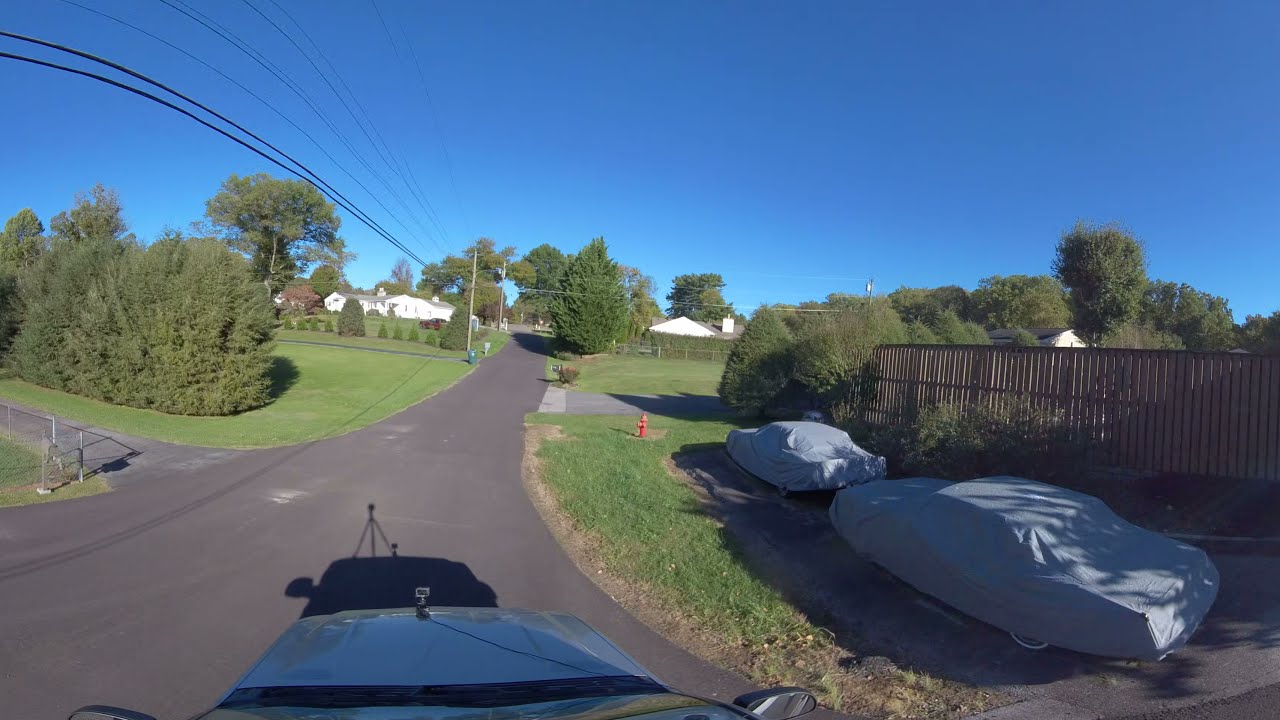The image captures a peaceful, residential neighborhood from the vantage point of a vehicle, possibly from the hood or the roof. In the foreground, the gray hood of the car, complete with a hood ornament and side view mirrors, is visible. The vehicle's shadow and a possible tripod-mounted camera suggest the image might have been taken within the car or attached to it.

Ahead lies a narrow, unmarked paved road extending through the neighborhood. On the right side of the road, two cars are parked with protective gray covers, one of which reveals a glimpse of a white wall tire. These vehicles sit in front of a fence lined with bushes, beside a prominent red fire hydrant. Following the fence, a yard transitions to another building, flanked by more shrubbery and a touch of greenery.

On the left side of the road, a driveway leads to a spacious yard bordered by purposefully planted trees. Power lines stretch overhead against a backdrop of a clear, blue sky, devoid of clouds. The entire scene is distinctly suburban, marked by neatly maintained lawns and driveways defining neighboring properties.